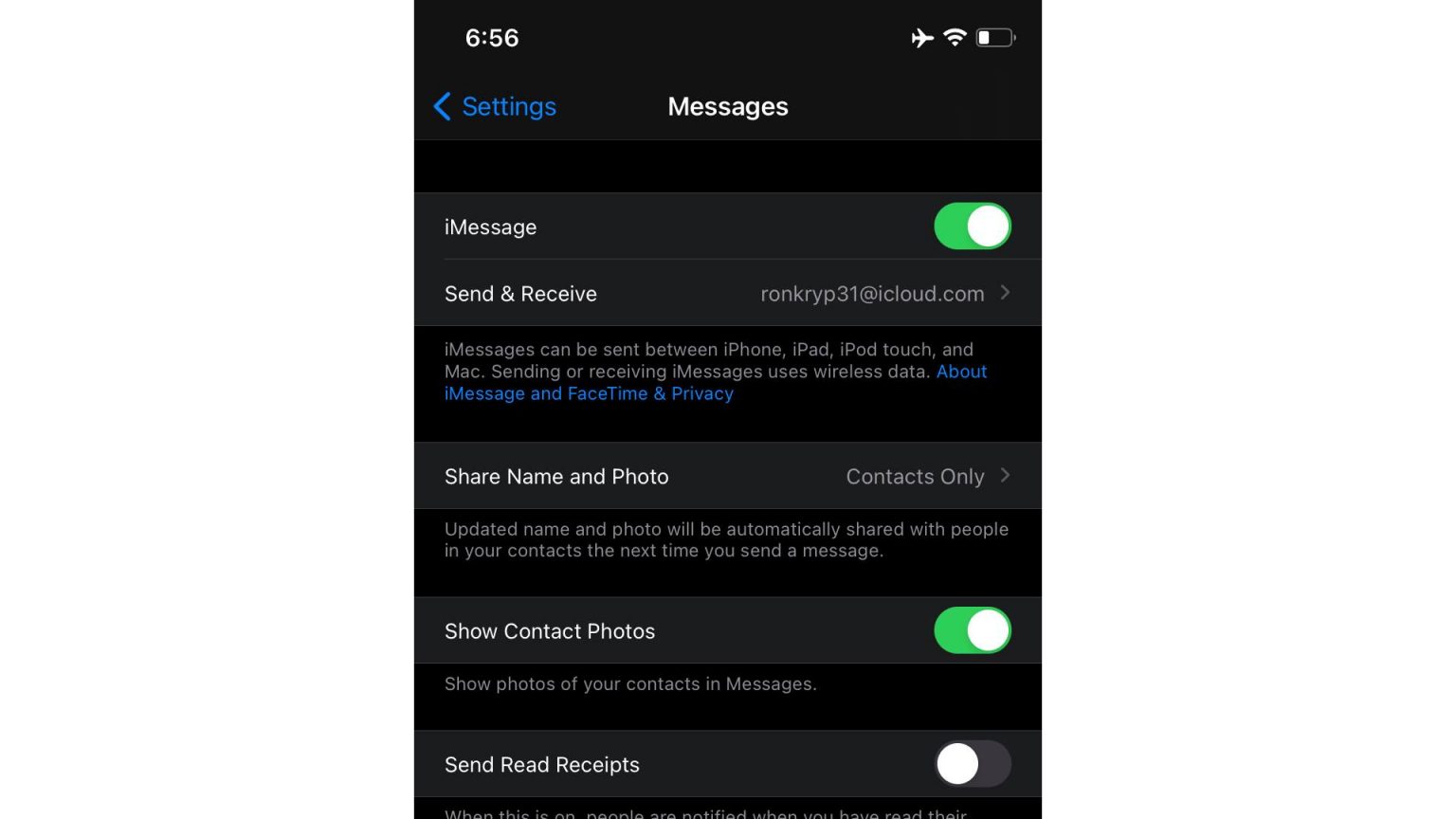The top-left corner of the screen displays the time "6:56". The background is entirely black. In the top-right corner, several status icons are visible: an airplane mode symbol, a Wi-Fi symbol, and a partially filled battery icon. 

Below that, the screen features a heading in blue text that reads "Settings" with a left-pointing arrow next to it. Beneath the heading, the text "Messages" is shown in white, followed by the label "iMessage". To the right of this label, there is a small green indicator.

Further down, the text "Send & Receive" appears, accompanied by the email address "wrong, gear 31 at icloud.com." Additional text notes that messages can be sent between iPhone, iPad, and iPod Touch. An informational section on "Sending and Receiving iMessages to this Wireless Terminal" is also present.

The text "About iMessage & Privacy", in blue, comes next. Below it, a gray dot precedes the option "Share Name and Photo", which is set to "Contacts Only". Additional text explains that updated names and photos will be automatically shared with people in your contacts using iMessage.

Another section titled "Show Contact Photos", indicated by a green switch, includes white text stating, "Show photos of your contacts in messages." Further down, a gray dot followed by white text reads, "Send Reader Receipts," next to a white circle toggle.

The overall theme of the screen is consistent with a settings menu, featuring a black background with various texts and symbols in gray, white, and blue colors.